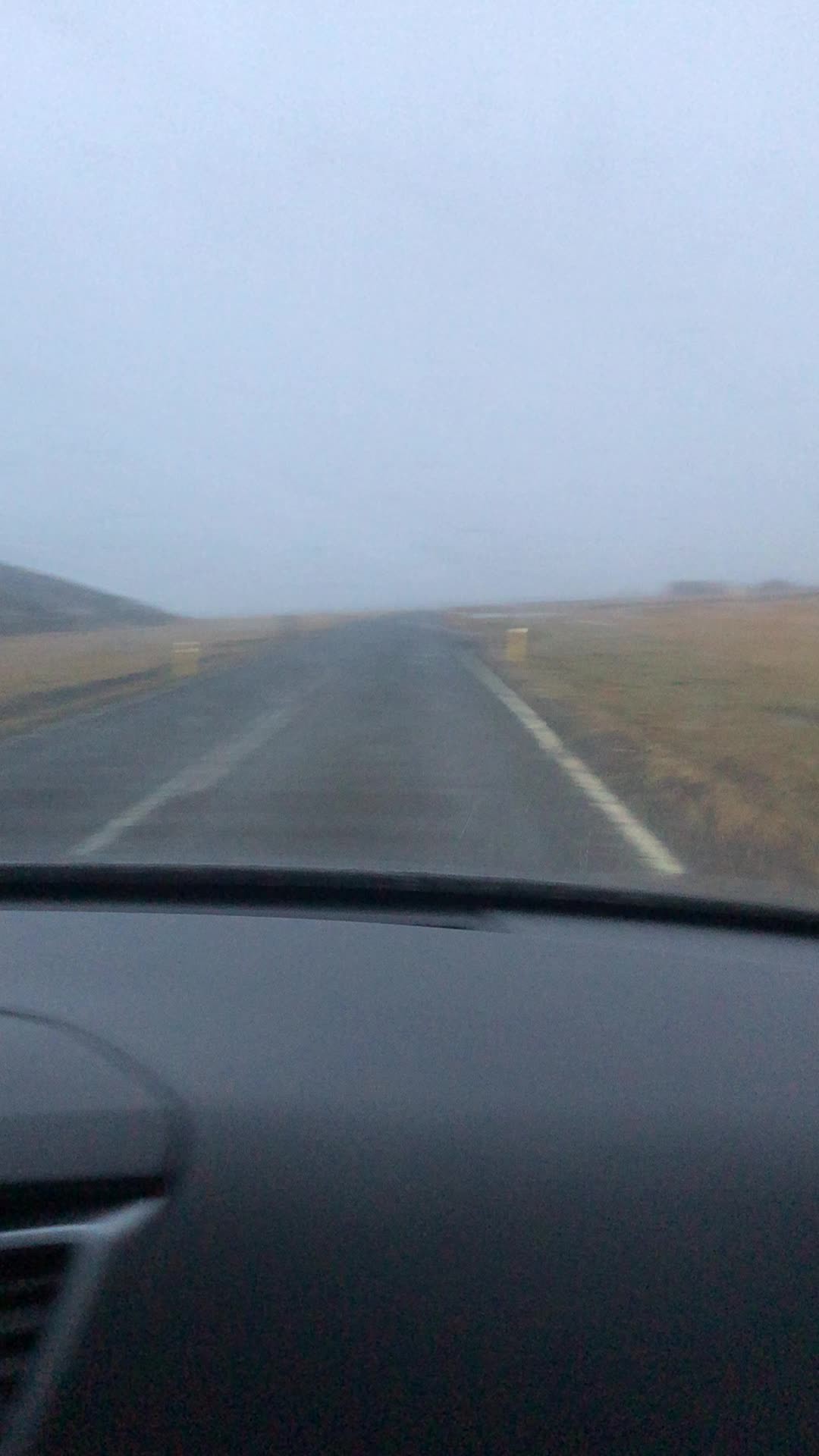The image is a blurry and foggy photograph taken from inside a car, capturing a misty and clouded road ahead. Shot through the windshield, the photo reveals a straight, black road with white lines, bordered by flat areas of prairie grass in browns, beige, and a bit of green. On the left side, a light brown barrier wall prevents cars from veering off, while further left, part of a low hill or mountain is visible. The sky is a light grayish-blue, entirely overcast with no clear visibility due to the fog. Inside the car, the dark dashboard is visible alongside an air conditioning vent, suggesting the photo may have been taken by a passenger on an older device, given the low image quality.